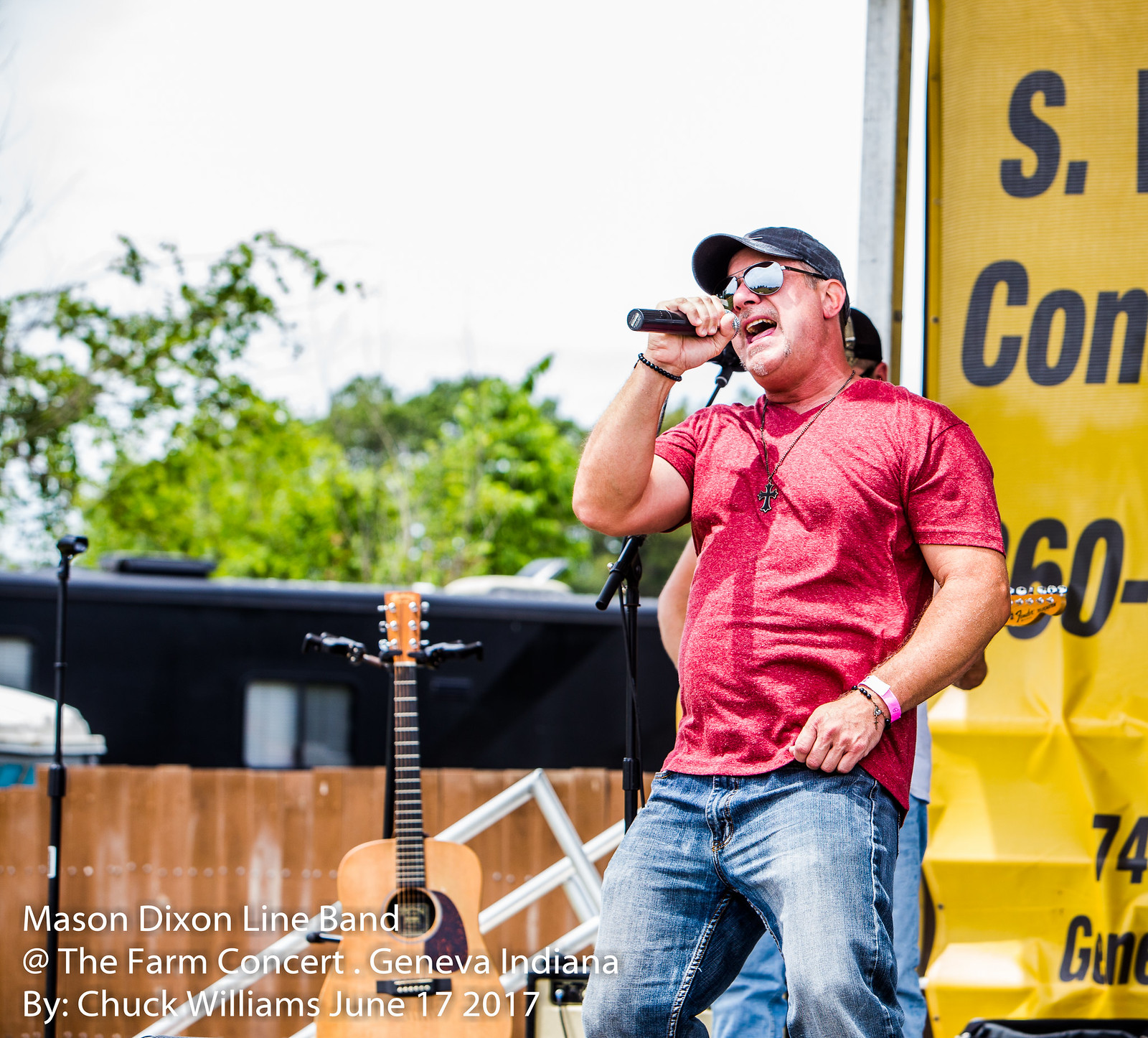The image is a detailed color photograph, oriented in landscape, capturing an outdoor stage performance. The focal point is a white male singer positioned prominently on the right, wearing a red t-shirt, blue jeans, dark sunglasses, and a black baseball cap. A cross necklace adorns his neck, and he's gripping a black cordless microphone close to his open mouth, revealing his teeth and tongue. He sports bracelets on both wrists, one resembling a charm bracelet. Behind him, slightly to the left, another man plays a guitar, and an acoustic guitar rests on a stand between two microphone stands. The backdrop features a wooden fence, a dark RV, trees, and a gray to light blue sky. To the right of the singer, a large yellow vertical banner with partially readable black text is visible. Small white text in the lower left corner reads: "Mason Dixon Line Band, at the Farm Concert, Geneva, Indiana, by Chuck Williams, June 17, 2017."